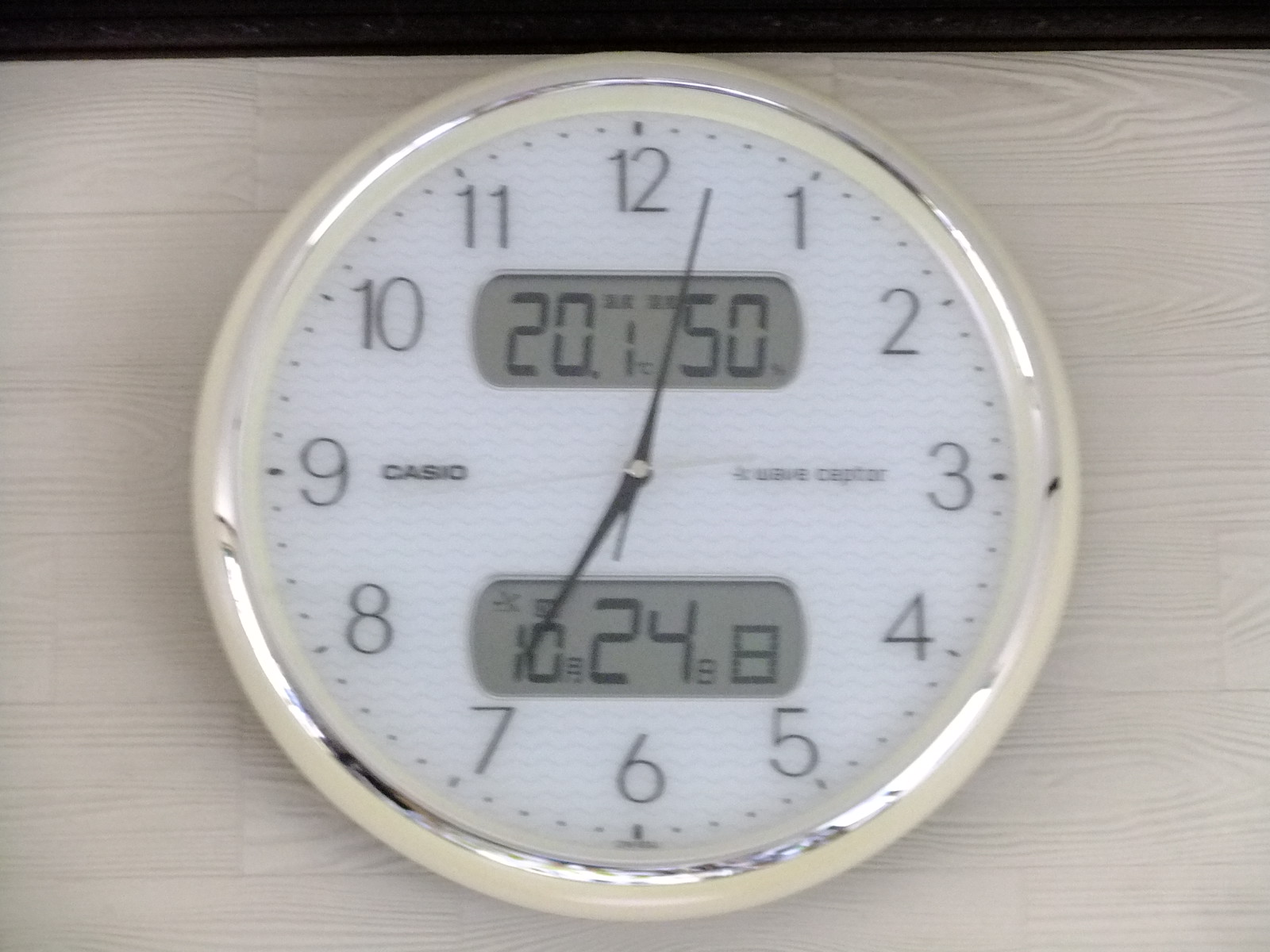This image features a Casio wall clock, prominently displayed against a white wood surface, which could either be a wall or a floor. The clock has a clean, white face, with standard numerical markings circling from 12 at the top to 11. Two distinctive, pill-shaped digital displays are incorporated within the clock's design. Although the photo is slightly out of focus, making details harder to discern, the upper digital display reads "20.1," likely indicating the temperature in Celsius. The purpose of the lower digital display remains unclear due to the image's quality but may be related to humidity or another environmental metric. The brand name "Casio" is clearly visible on the clock's face, emphasizing the clock's reputable maker.